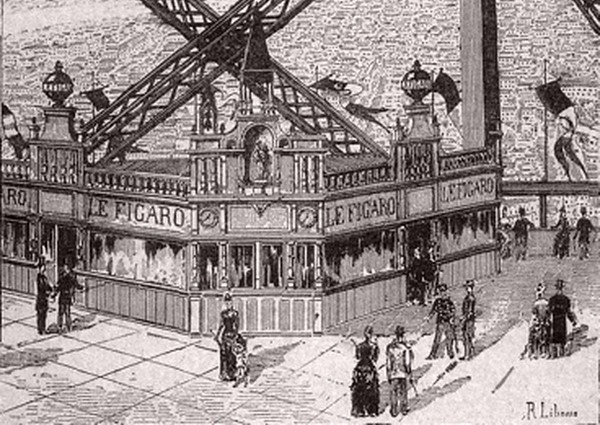This black and white illustration, potentially drawn with pen or pencil, captures an old-fashioned street corner scene from the late 18th to early 19th century. The focal point of the image is a one-story corner store named "Le Figaro," prominently displayed in bold lettering on light-colored rectangles above wide windows. The storefront's architecture is accentuated by steel girders crisscrossing at the top, extending left and right, possibly part of an overhead structure. 

The image features various pedestrians—men in suits with top hats and women in corset-style, long-sleeved dresses—conversing and walking in front of the store's multiple entrances. The scene is busy with about half a dozen people spread throughout the sidewalks and crosswalks situated at the bottom portion of the image. In the background, a city landscape stretches out, adding depth to the setting. Distantly, the scene hints at either a natural landscape or waterfront beyond a railing, accented with a couple of flags.

The detailed craftsmanship is signed at the bottom right by the artist, with a barely legible signature reading "R-L-I-B-E-N-E-S."